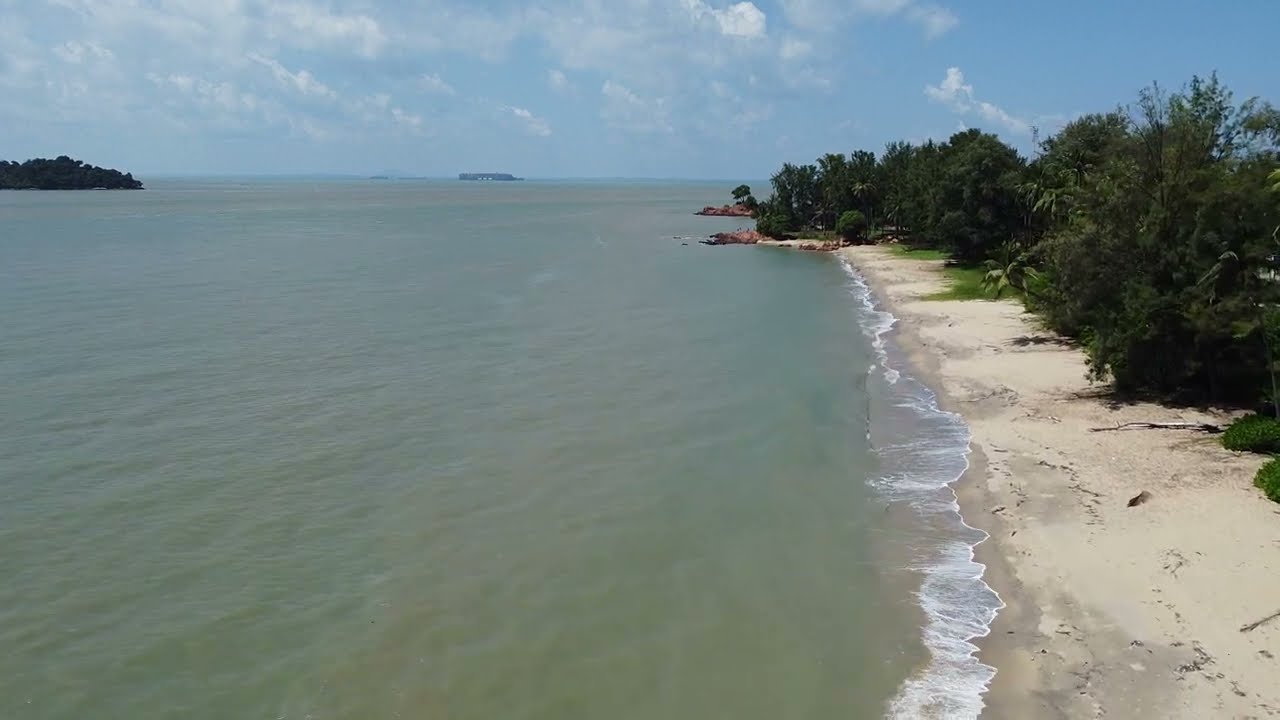The image depicts a secluded, rugged beach scene without any text, people, or animals present. On the far right side of the image, a sandy embankment extends vertically, bordered by several tall green trees and bushes. These trees stretch towards the sky, which occupies the top quarter of the image and is a blend of light blue and white, dotted with a few puffy clouds. The left side of the image is dominated by a large body of water with light waves crashing gently onto the sand. This water is light greenish-brown in color and occupies most of the frame. In the distant background on the left side, there's a hint of what appears to be an island or possibly a structure, such as a cargo ship, further emphasizing the remoteness of the setting. The entire scene exudes a sense of calm and solitude, with no visible sun, suggesting it might be taken in the middle of the day.